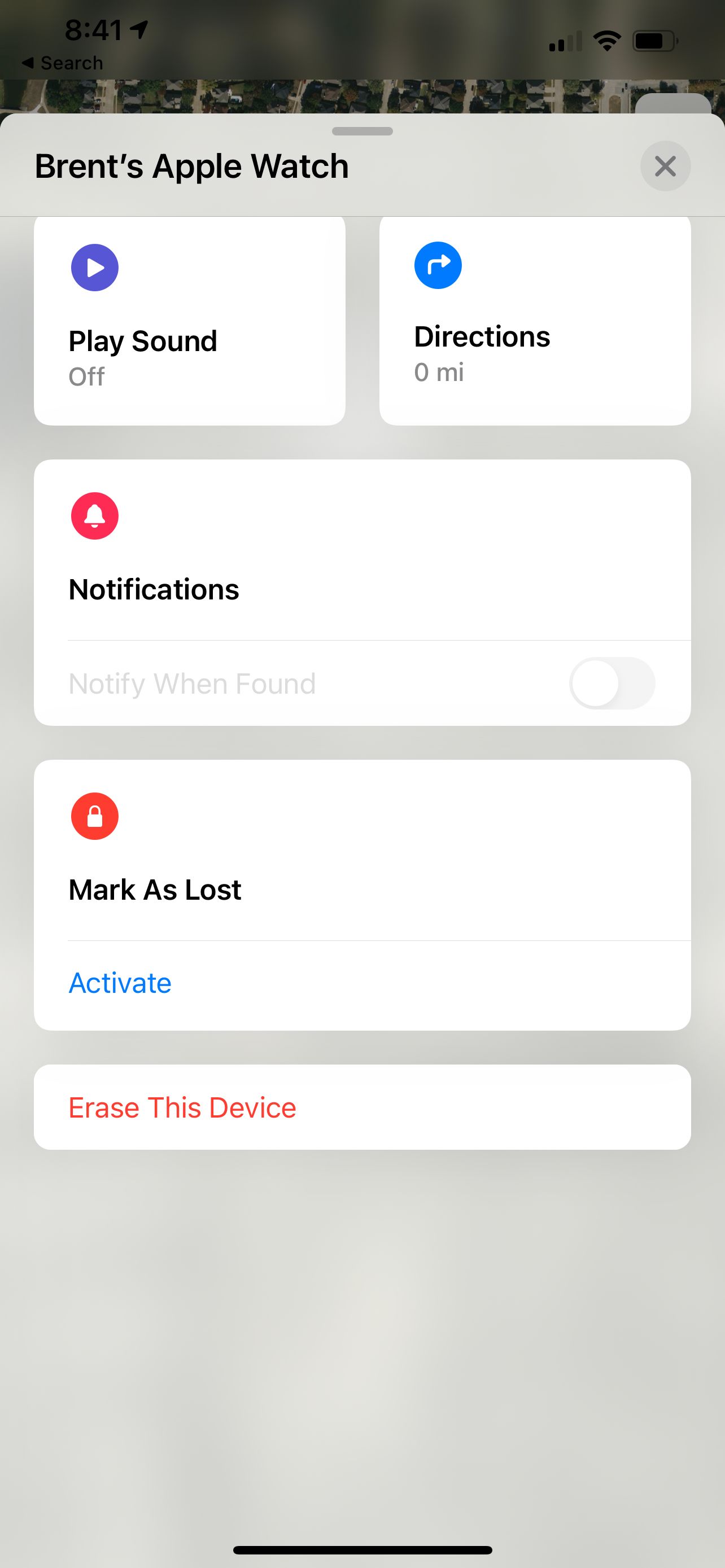The image displays a digital interface on a dark grey background, indicating the time at 8:41. The display shows the device has 2 out of 4 bars of signal strength and approximately three-quarters of battery life remaining.

Below this, the screen features a grey section titled "Brent's Apple Watch" with an 'X' icon to its right. Underneath, there is a white box with a blue circle containing a play button, labeled "Play Sound Off." To the right, another white box with a blue circle and a right-pointing arrow is labeled "Direction, 0 miles."

Further down, there is a white rectangle with a red circle and a white bell icon, accompanied by black text that reads "Notifications." A grey line separates this from another option titled "Notify When Found," which has a switch turned to the left, indicating it is off.

Another section features a white rectangle with a circle and a lock icon labeled "Mark as Lost," with a blue hyperlink that says "Activate." At the bottom of the display, in red text, it reads "Erase This Device."